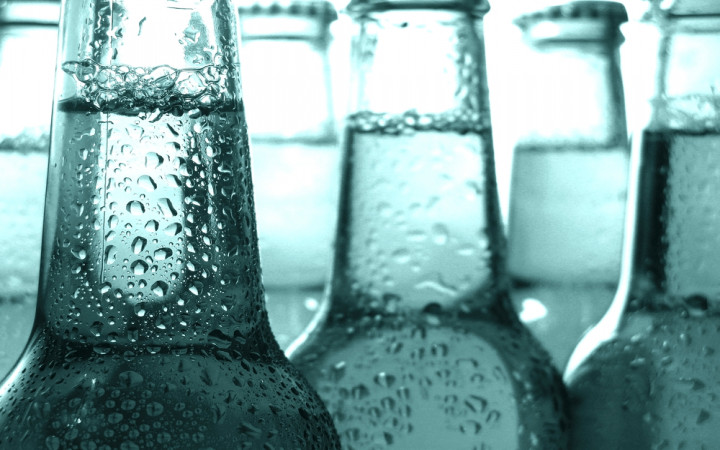A close-up photo showcases six blue-tinted glass bottles filled with clear liquid, reaching up to the neck. Each bottle has a silver twist-off cap and stands upright, with visible condensation and sweat marks on the exterior. The bottles are arranged in slightly different rows, with one bottle closer to the camera. The background of the image is brightly lit, possibly by sunlight, which creates a shine on the bottles. One noticeable feature is the presence of a white, heart-shaped object inside one of the bottles. The first bottle on the left is slightly darker as it's not directly illuminated. All bottles remain unopened and fully filled.